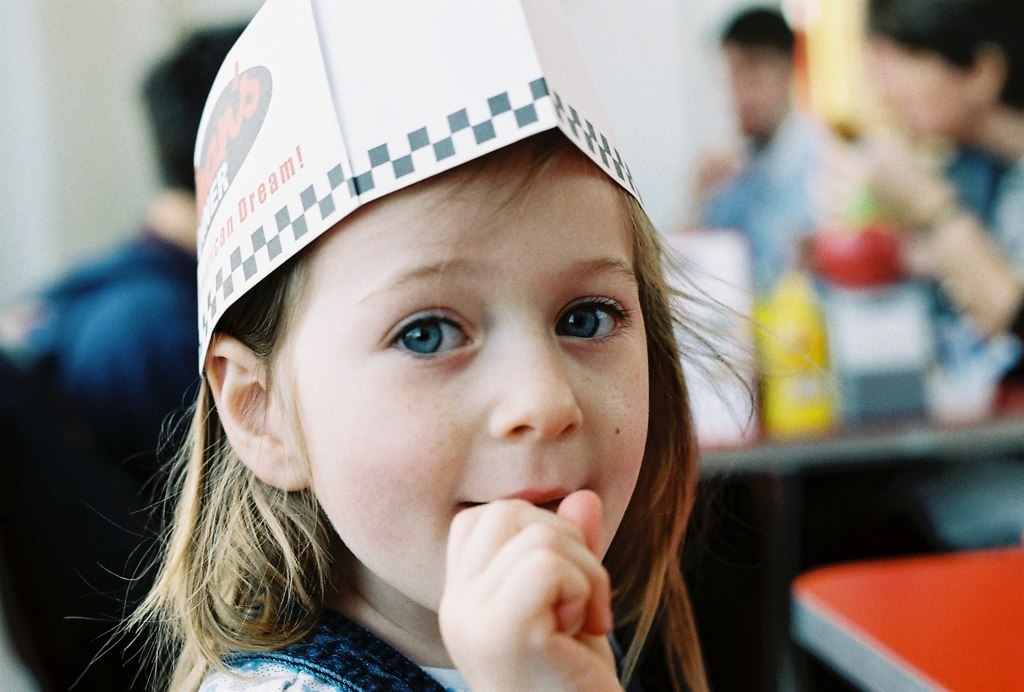In this photograph, a young girl, appearing to be around six or seven years old, sits in what looks like a fast-food restaurant or diner. She is a white female with blonde hair and strikingly large blue eyes. She is wearing a promotional paper cap, likely from the restaurant, which features a black and white checkerboard pattern along the bottom edge and the phrase "Ken Dream" with partially visible letters "ER" on the logo.

The girl is dressed in blue overalls paired with a white shirt and has her right hand in or near her mouth. She gazes directly at the camera, appearing contemplative or curious. Behind her, the setting is filled with diners; three indistinct figures are seated at tables, engaged in eating, and the background appears blurry.

More detailed observations reveal a yellow mustard container, a red item (possibly an apple or a ketchup bottle), and a napkin holder placed on the table behind her. The dining table surfaces are orange or red, and one of the blurry figures in the background seems to be wearing a backpack and a blue shirt, adding to the casual, everyday atmosphere of the scene.